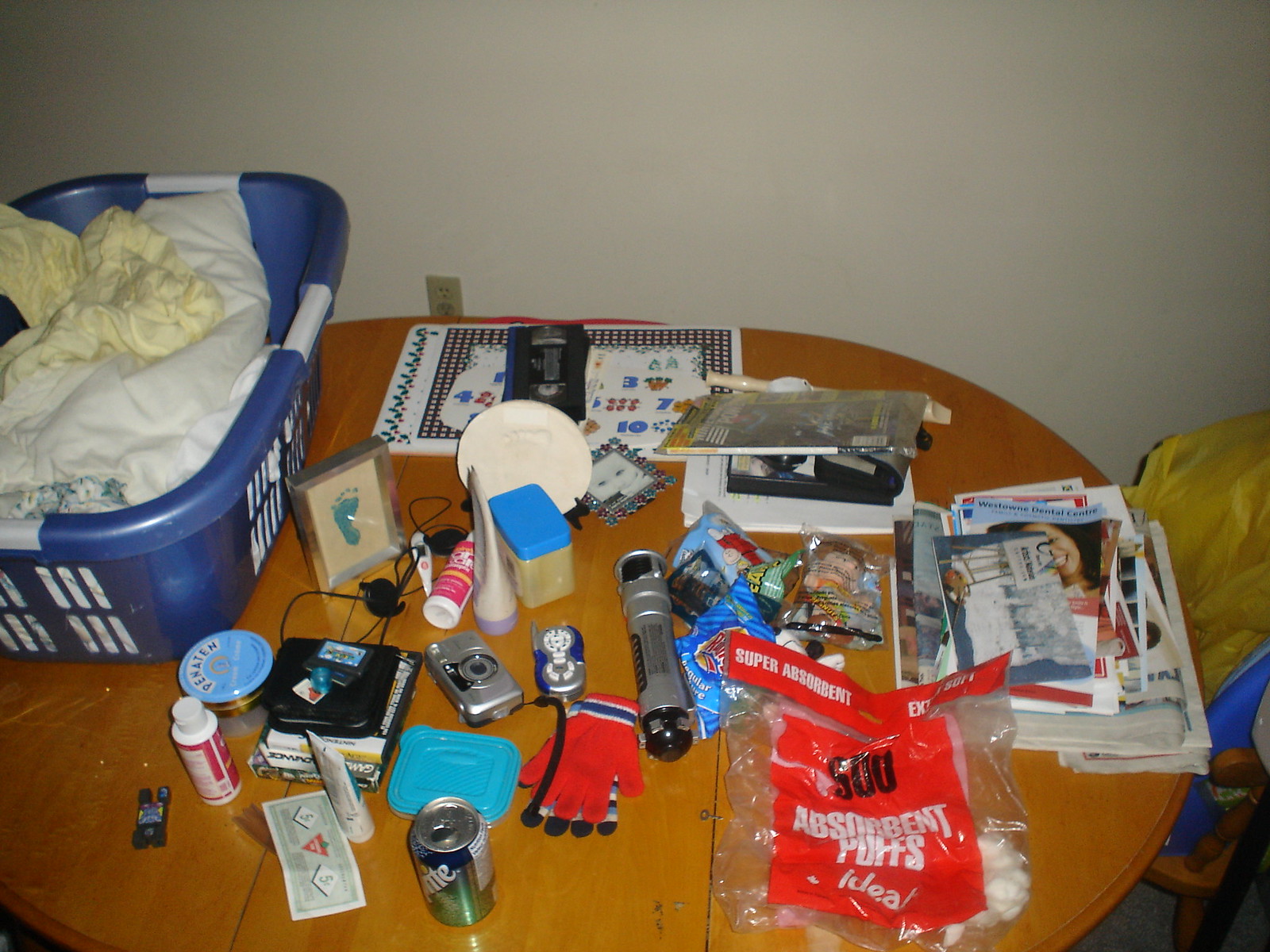The image presents a three-piece wooden table viewed from a diagonal, top-down angle. The table occupies most of the frame, extending slightly beyond the left edge, with a small gap visible to the right. Various items clutter the tabletop, painting a vivid picture of everyday life.

In the upper left quadrant, a portion of a blue laundry basket, partially obscured by about 25%, can be seen. It brims with white and yellow linens. Moving to the lower left corner, there are several bottles and tubes, accompanied by what appears to be fake money and an open can of Sprite. Nearby, the lid of a Tupperware container rests close to the table's center.

A digital camera lies near the middle areas of the table, where a red glove is draped over a multicolored rainbow glove. Beside these, a lightsaber hilt inscribed with text can be spotted. In the lower right section, a bag of absorbent puffs or cotton balls is noticeable. Further to the right, the table becomes a repository for reading materials, with magazines and newspapers stacked in the center-right area.

Toward the center af the table appears a jar of Vaseline, while an upper central spot features a placemat, adding a touch of order to the otherwise eclectic array of items.